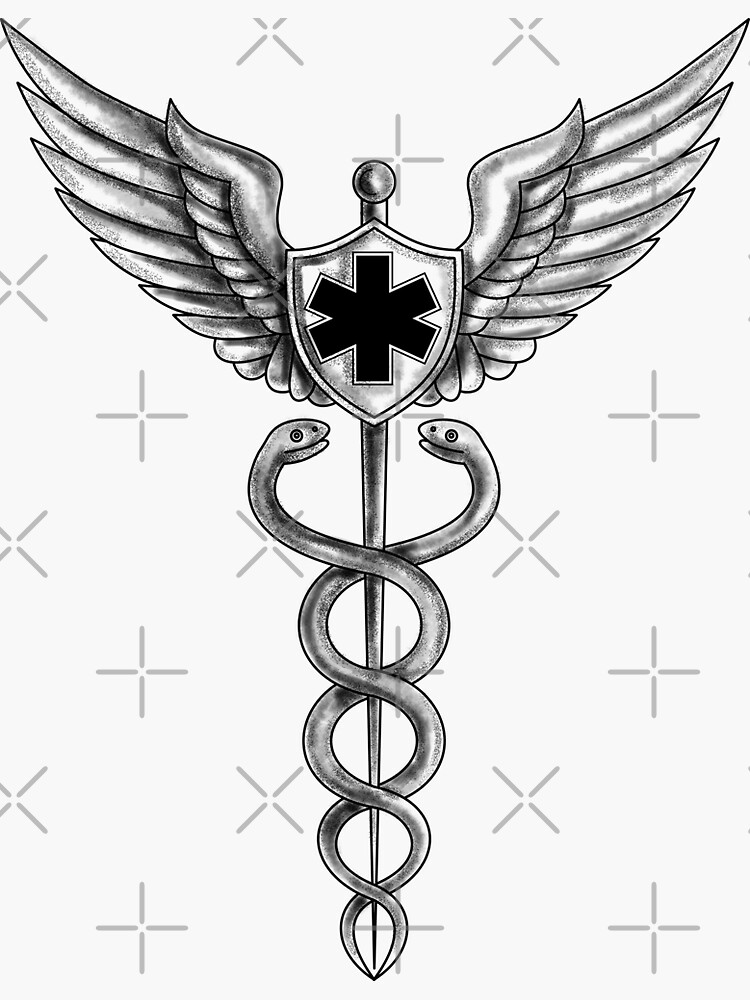The image is a detailed pen and ink illustration, accented with pencil shading, primarily in black and gray tones. It features a staff that, while reminiscent of a caduceus, incorporates unique elements suggesting a military medical emblem. The central staff, which tapers towards the bottom where the intertwined snakes' tails end, is adorned at the top with a round pommel. A prominent shield is positioned at the upper part of the staff, emblazoned with a thick-lined, six-pointed cross—resembling a sideways 'X' intersected by a vertical line. Surrounding this shield are two sets of wings that extend outward, with an intricate layering of feathers: a shorter tier closest to the shield and a longer tier extending further out. The heads of the snakes wrap around the staff, facing towards each other with their mouths slightly open. The background is white, scattered with cross and X watermarks, giving the appearance of a transparent, clip-art style setting. The entire illustration stands as a symbolic representation of health, commonly associated with medical personnel, including doctors, nurses, and military medics.